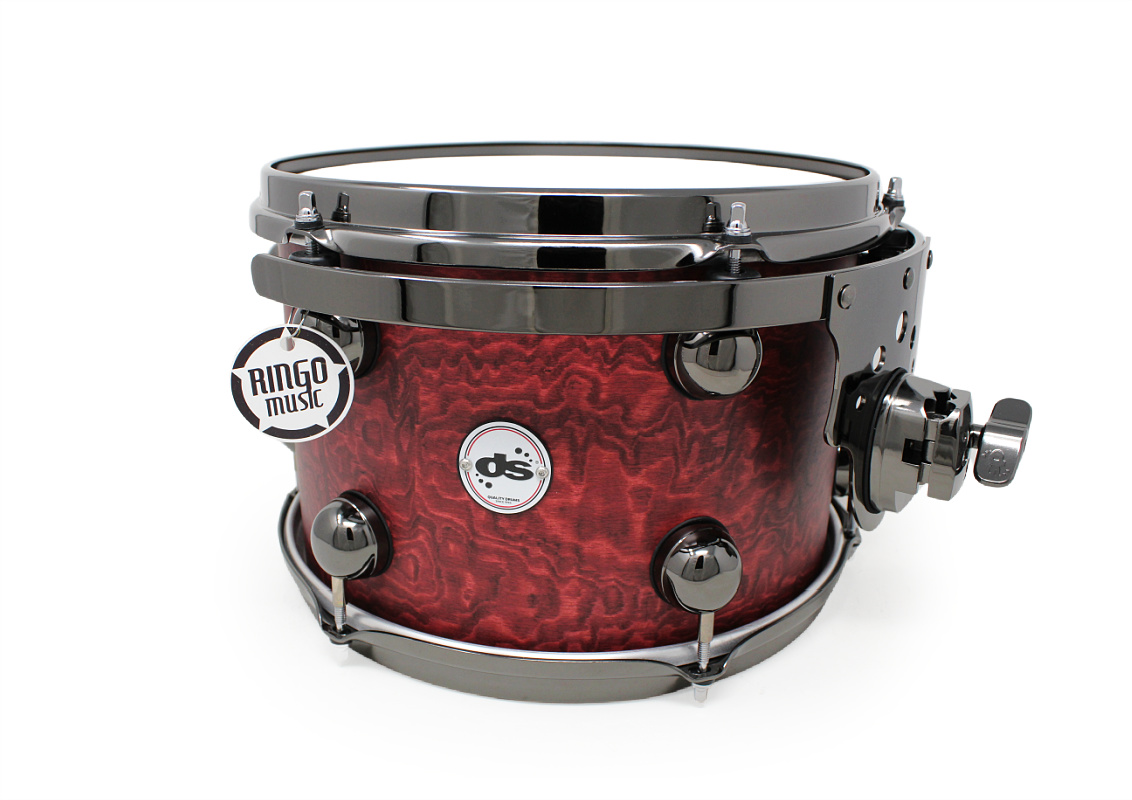This image showcases a close-up of a single drum, likely a snare drum or tom-tom, set against a plain white background. The drum features a striking maroon to reddish body adorned with a swirling pattern of black and gray accents. Its top surface is white, held taut by a shiny, silver-gray metallic rim, bolstered by several turn screws that secure the top to the body. Prominently displayed on the drum is a circular logo that reads "DS," encircled by a red and blue ring, with dots arranged in a circular pattern around the letters. To the left, there is a hang tag in a white spiked circle edged with black, inscribed with "Ringo Music" in bold black letters. The drum is fitted with a silver handle on its right side, possibly used for tuning or adjustments. The entire drum appears new, with its metal components gleaming and reflective, adding to its overall polished look.